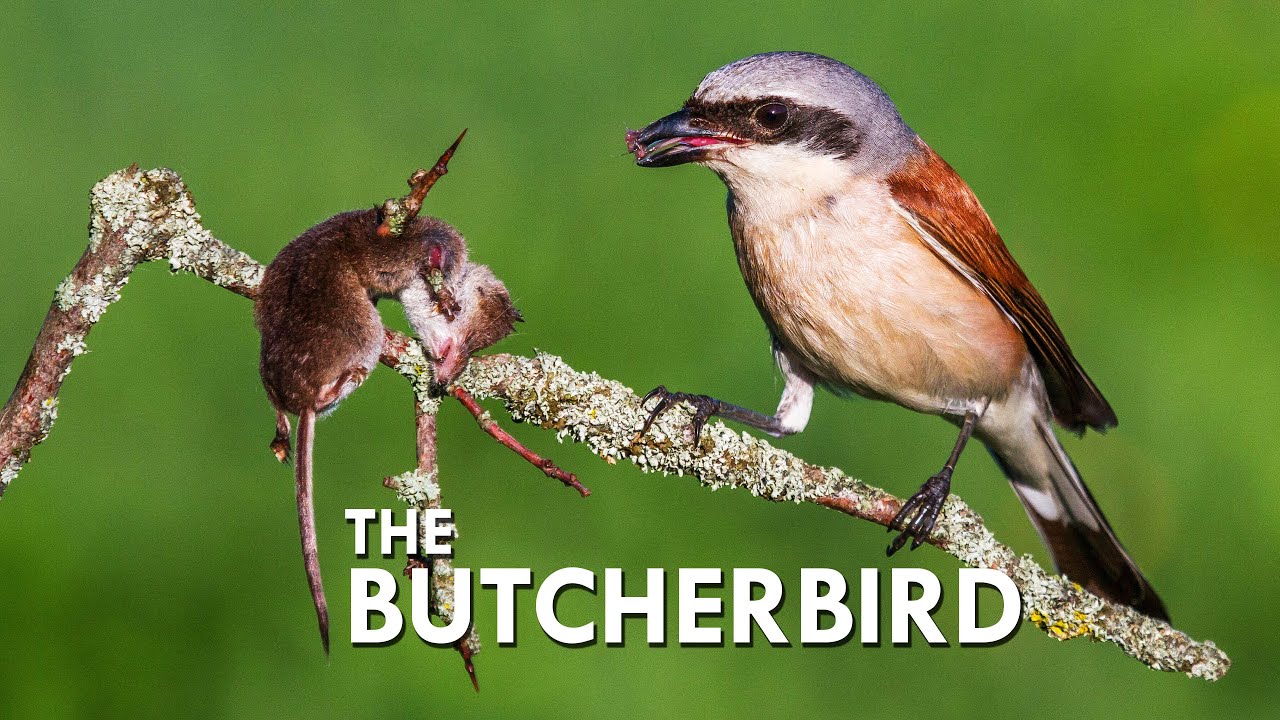The photograph, oriented horizontally, captures a striking scene of a bird perched on a tree branch with a blurred backdrop of green grass or bushes, which directs focus onto the bird and its prey. The bird, identified by the white text "The Butcher Bird," features predominantly brown feathers on its back, a white tan underbelly, and a white head with an olive green streak around its eyes. It has small black eyes and a dark beak, from which a bloody piece of meat dangles, indicating it has begun its meal. The bird's tail is a darker brown, and its wings exhibit a mix of grayish and brown tones.

In front of the bird, impaled on a thorny branch, is a small rodent, most likely a mouse, showcasing signs of a violent end with visible blood and damaged fur. The mouse's body is brown with patches of white, impaled and slouched, evoking the bird's gruesome hunting technique that earned it the name "Butcher Bird." This detailed and graphic depiction underscores the bird's predatory nature and creative method of handling its prey.